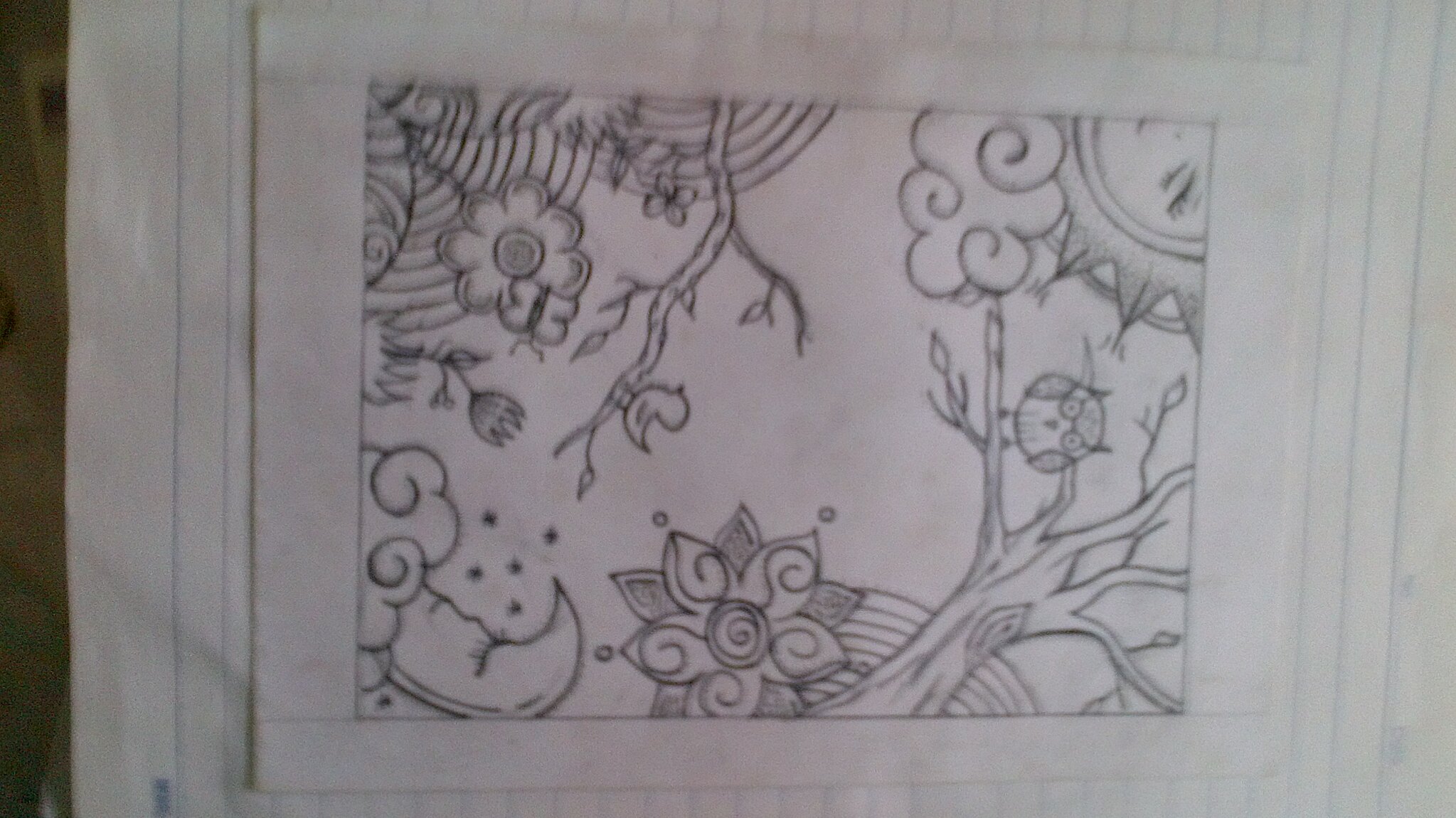This detailed black-and-white illustration captures a whimsical fairy tale scene. At the bottom of the image, a leafless tree stands, its barren branches winding skyward. Perched on one of the limbs is a simplistically drawn owl, with a round body and large, expressive eyes. To the right of the tree, a radiant sun with a serene, smiling face and closed eyes adds a touch of warmth to the composition. On the lower left side, a crescent moon, depicted in profile with shut eyes and a peaceful expression, enhances the mystical atmosphere. Above the moon, a delicate branch extends from what seems to be a field of flowers, supporting a small bird poised calmly. The entire scene evokes a sense of tranquility and enchantment, reminiscent of classic fairy tale illustrations.